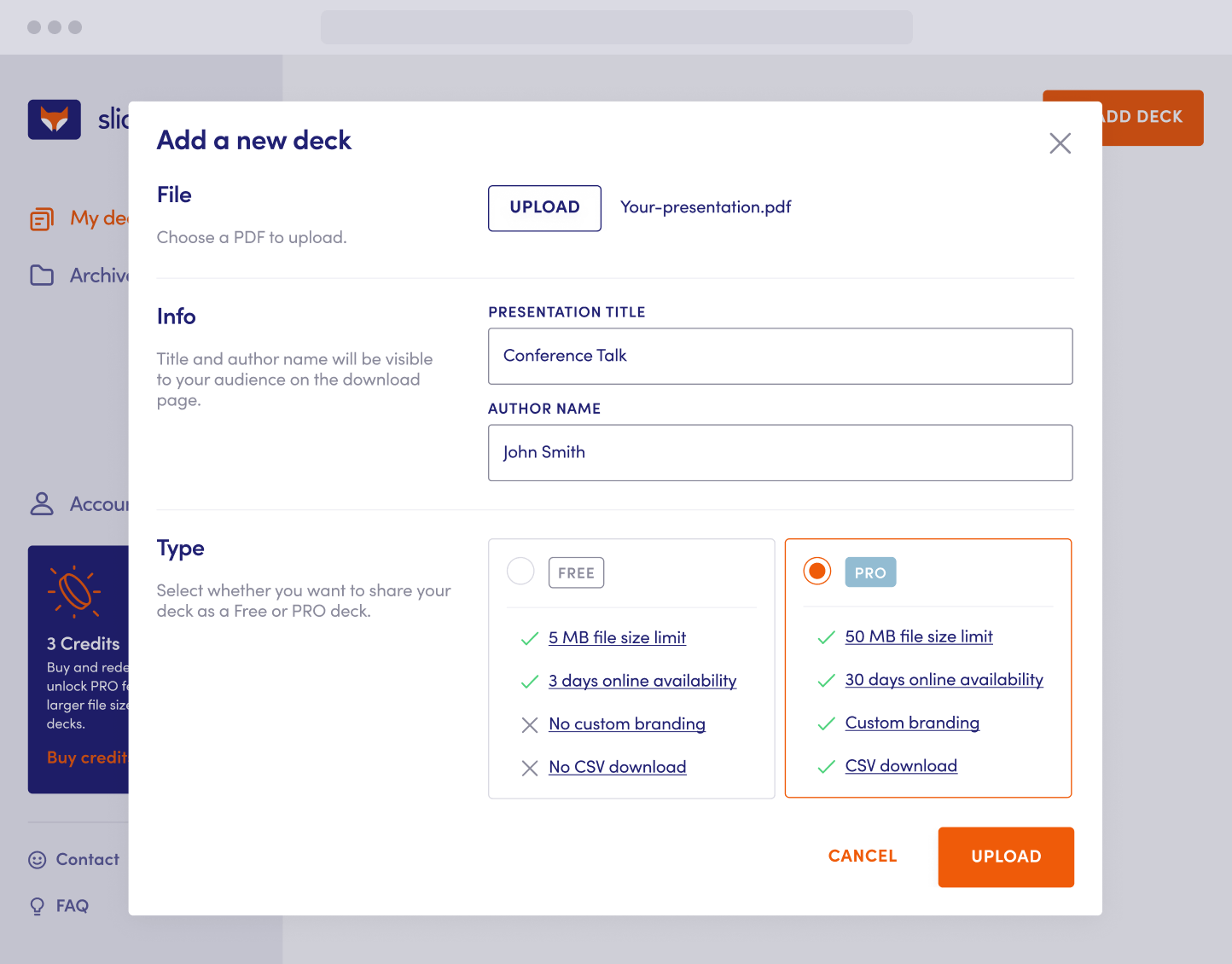This image appears to be a screenshot of a webpage featuring an active pop-up dialogue box. The pop-up box is white with blue and black text and is situated against a greyed-out background. In the backdrop, there are three dots in the upper left-hand corner, a search bar, and a logo that resembles the head of a fox with a red top and white bottom, marked with "S-L-I" in blue text next to it. Below the logo, some orange text reads "MYDE", followed by an archive account box indicating "three credits" with an icon of a phone situated within a blue box. To the right side of the background, a fragment of an orange checkbox with partial white text displays the letters "deck".

The pop-up dialogue box itself bears the title "Add a New Deck" in its upper left-hand corner. It provides an interface for uploading a presentation PDF, with a "File choose a PDP to upload" field and an accompanying "Upload" button on the right. Detailed instructions state that "title and author name will be visible to your audience on the downloaded page." Fields for "Presentation Title" and "Author Name" are visible, with "Conference Talk" and "John Smith" entered, respectively. 

Further, the pop-up explains options for how the deck can be stored under a section labeled "Type." Users can choose to store their deck as either "Free" or "PRO." The "Free" option allows 5 megabytes of file size, 3 days of online availability, no custom branding, and no CSV download. The "PRO" option, which is currently selected, allows 50 megabytes of file size, 30 days of online availability, custom branding, and CSV download. At the bottom right-hand corner of the dialogue box, there are "Cancel" and "Upload" buttons, with the "Upload" button in orange, ready for action.